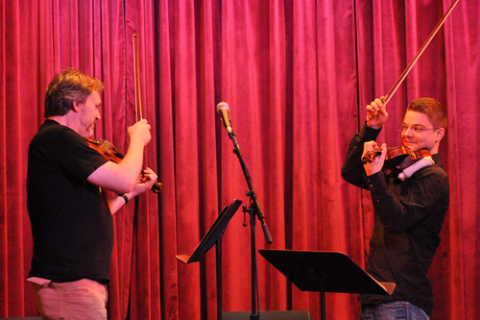A middle-aged man and a teenage boy, possibly a father and son, are playing a lively duet in front of a luxurious red velvet curtain. Both have sandy hair, with the teenager sporting glasses. The man appears to be in his mid-40s and wears a long-sleeved black shirt, while the teenager, likely between 15 and 17 years old, wears a short-sleeved black shirt. They each hold violins, propped against their chins, and bows, though one bow seems noticeably longer than the other. Their music stands, positioned at waist level, may or may not hold sheet music, given their angles. A single microphone is set up between them to amplify their performance. The man on the left, who has a watch on his left wrist, and the boy on the right are both smiling at each other, hinting at a joyful connection through their fast-paced musical piece.